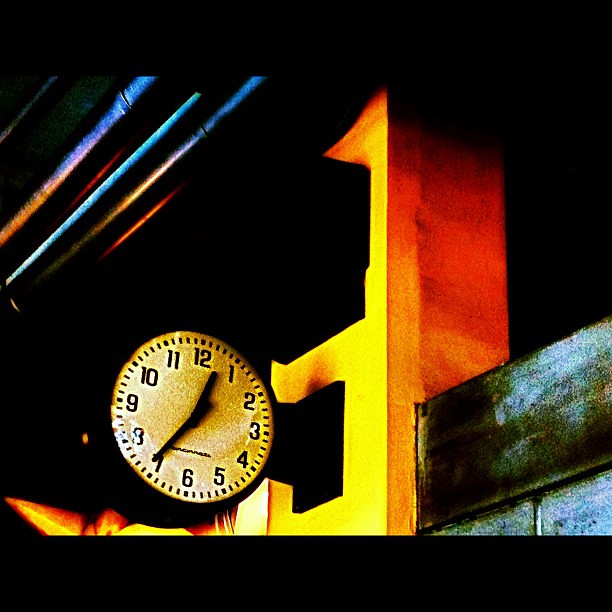The image showcases a white-faced wall clock with black minute and hour hands, displaying the time as 12:36. The clock is mounted on its right-hand side by a black bracket, connecting it to a tall, yellow structure that spans the entire height of the frame. To the left of the clock, three vertical pipes hang, extending from the left middle side to the top left corner of the photograph. To the right of the yellow structure, there is a gray cinder block fixture. At the bottom of the image, a black band serves as a framing element, adding contrast to the composition.